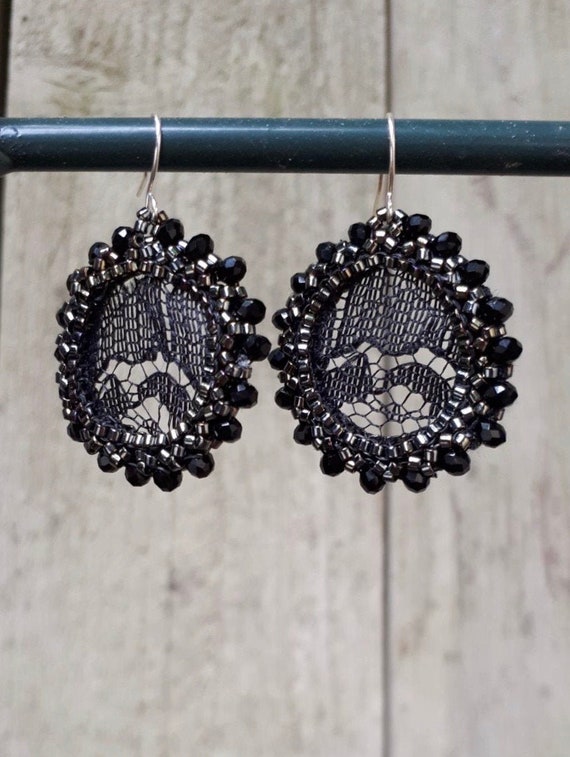The image showcases a pair of intricate, circular earrings hanging from a thin, plastic blue rod positioned in the foreground. The earrings, designed for pierced ears, feature silver hooks. They appear lightweight and are characterized by their unique artistry. Each earring forms an elegant oval or circular shape with an outer ring adorned with tiny, dark—almost black or purplish—globes, possibly small beads or gemstones. This outer ring also includes additional small silver beads. 

The center of the earrings is detailed with a complex web-like design that could resemble an abstract embroidery or a woven scene, possibly depicting mountains or resembling a spiderweb. This inner pattern varies slightly in density, with the top portion appearing more densely woven than the bottom. The background is deliberately out of focus, showcasing a wooden wall with a visible wood grain pattern and gray slats, emphasizing the earrings as the primary subject of the photo.